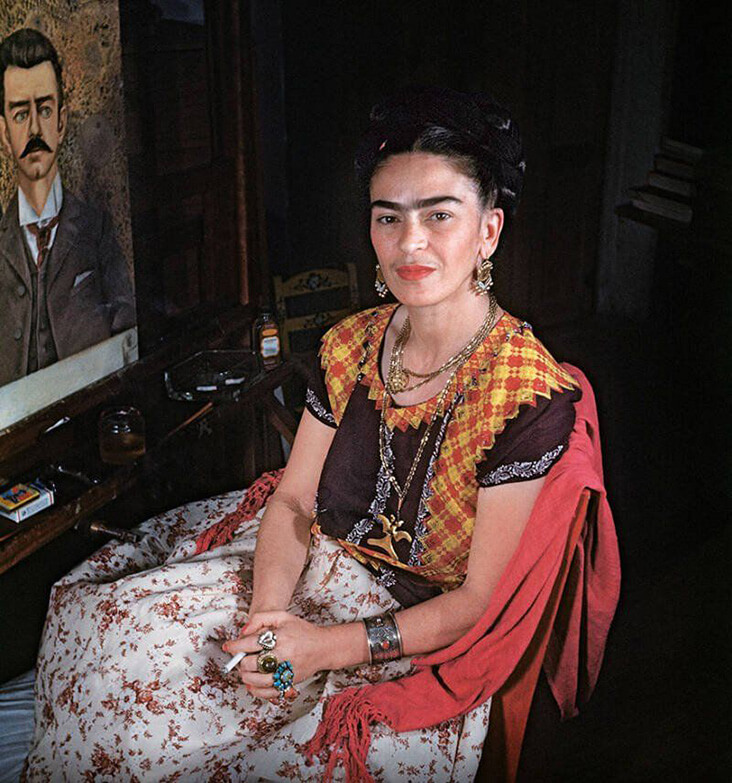In the square picture, we see a Mexican woman sitting and staring directly at the camera, offering a slight smile. She has dark hair that is put up and noticeable, very long brown eyebrows. She accessorizes with large, gold and diamond earrings and several rings adorning her left hand, alongside a thick metal bracelet on her left wrist. The woman dons a patterned top featuring shades of brown, orange, and red, paired with a floral skirt in similar hues, displaying white, brown, and red flowers. She also wears a couple of silver necklaces. In her left hand, she holds a cigarette. 

A red blanket or shawl drapes over the back of her chair. To her left, there is a painting above a shelf or table filled with what appears to be art supplies. The painting is a headshot of a man with a thick mustache, dressed in a brown suit paired with a blue shirt. The background behind her is dark wood, enhancing the rich tones of the setting.